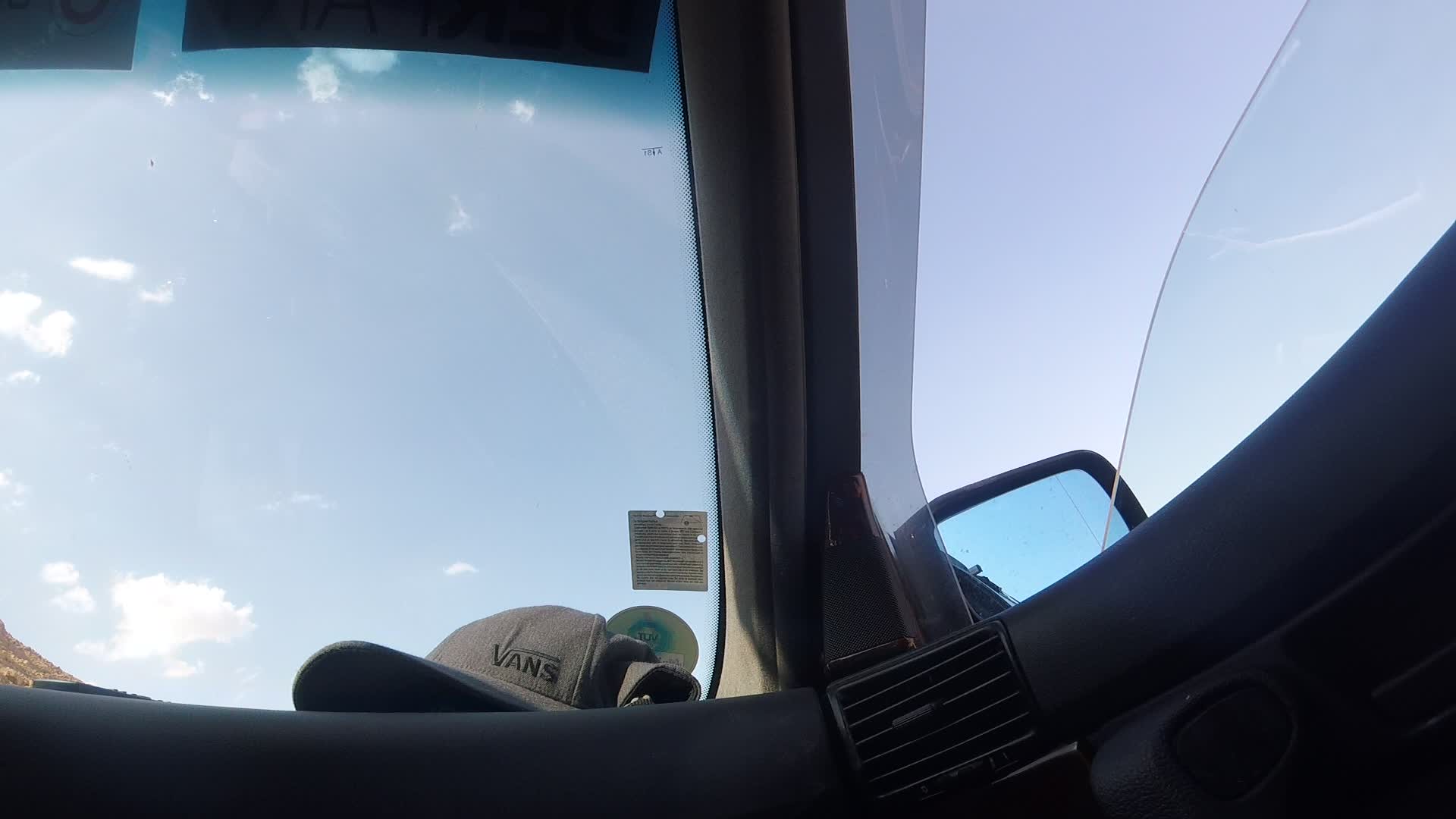The landscape-oriented color photograph is taken from inside a vehicle, capturing an upward 45-degree-angle view through the front windscreen and the right front window. The bottom of the image features a section of the black dashboard, arcing slightly from the bottom left towards just off the center to the right, showcasing a typical horizontal car air vent with visible plastic horizontal fins. Resting on the dashboard is a dark grey baseball cap with the brand name "VANS" written in black text on its side. 

The slightly down right front window reveals the half-lowered pane, curving mid-way through its open gap. Outside the window, the upper two-thirds of the wing mirror is visible, with a faint reflection of the vehicle’s body in its bottom left corner. The sky captured outside is light blue with a few scattered white clouds, indicating a sunny day. Additionally, the image shows the cream-brown support pillar at the vehicle's middle, providing structural strength for the windscreen. There are also multiple white stickers with dark writing visible on the windscreen and the top left corner of the image.